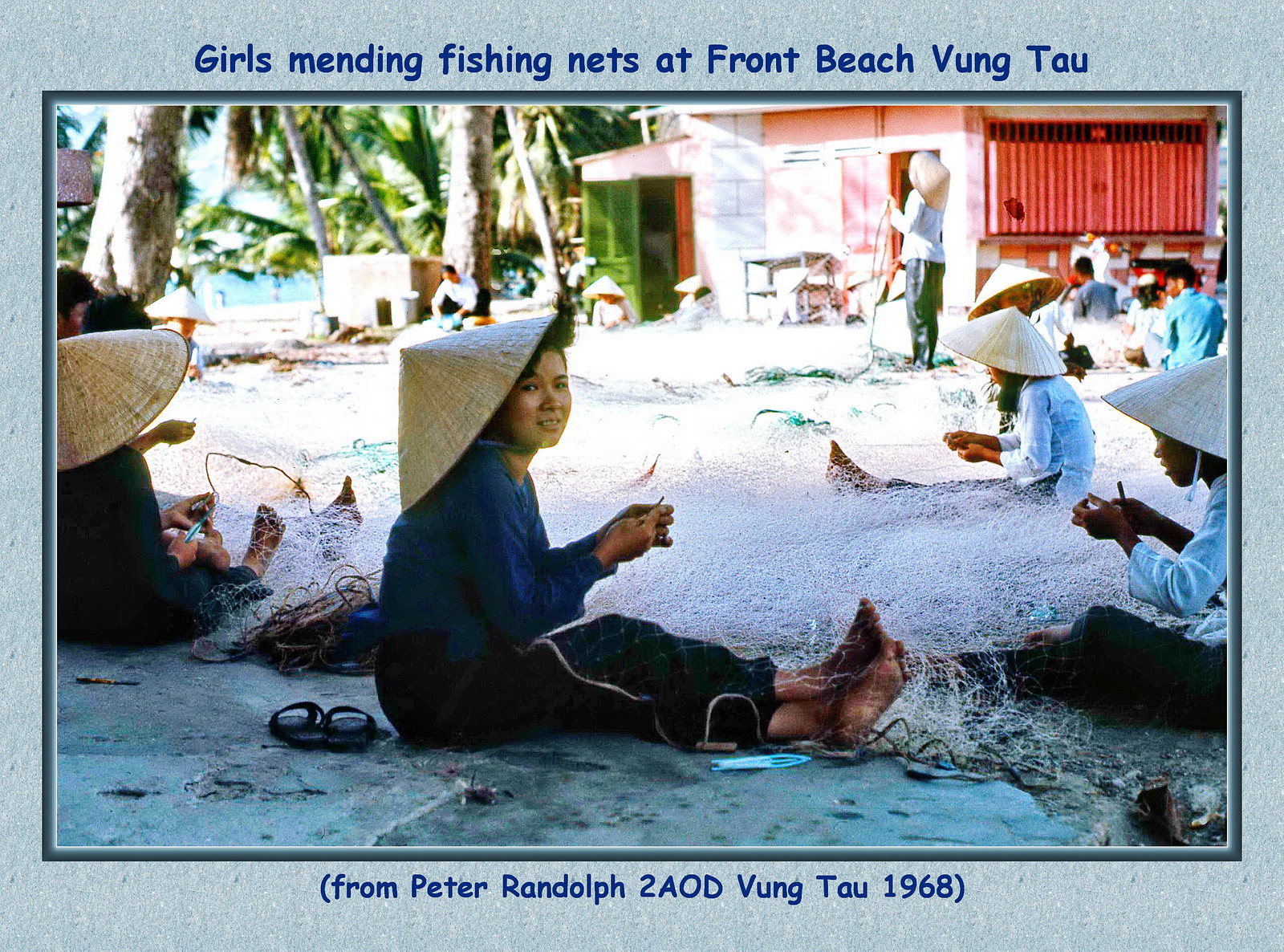In this image, we see a vibrant scene from an Asian country, specifically a snapshot of daily life in Front Beach, Vung Tau, captured in a 1968 postcard. The photograph shows a group of girls mending a large, white fishing net, seated on the ground and wearing distinctive straw hats that shield them from the sun. These girls are barefoot, focusing intently on their work, with an assortment of tools to fix the nets scattered around. Sunglasses lie on the ground nearby, adding a casual touch to the scene.

Behind the girls, on the left side of the image, a cluster of tall palm trees creates a lush green backdrop, while on the right, a red building stands out prominently. Some males are also visible in the background, near the building; unlike the girls, they are not wearing hats, and it is unclear if they are involved in mending the nets or just present.

The postcard is bordered in blue and features captions in blue text. At the top, it reads "Girls mending fishing nets at Front Beach Vung Tau," while at the bottom, a note from Peter Randolph to A0D Vung Tau adds a personal touch to the historical image. This detailed depiction offers a glimpse into the communal and labor-intensive aspects of life in Vung Tau during the 1960s, highlighting both the cultural attire and the shared workspace of the community.